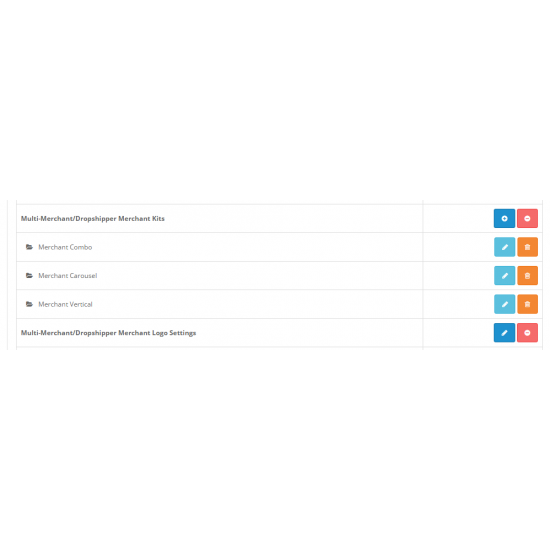Screenshot of an application interface featuring a section titled "Multi-Merchant Dropshipper Merch." The text is notably small and in a dark grey font on a white background, making it difficult to read. This section includes various options such as "Merchant Kits," "Merchant Combos," and what appears to be "Merchant Verticals." Below these options, additional text reads "Multi-Merchant / Dropshipper Merchant." To the right side of each option are two small buttons: a blue button with a pencil icon for editing, and a red button with a garbage can icon for deleting.